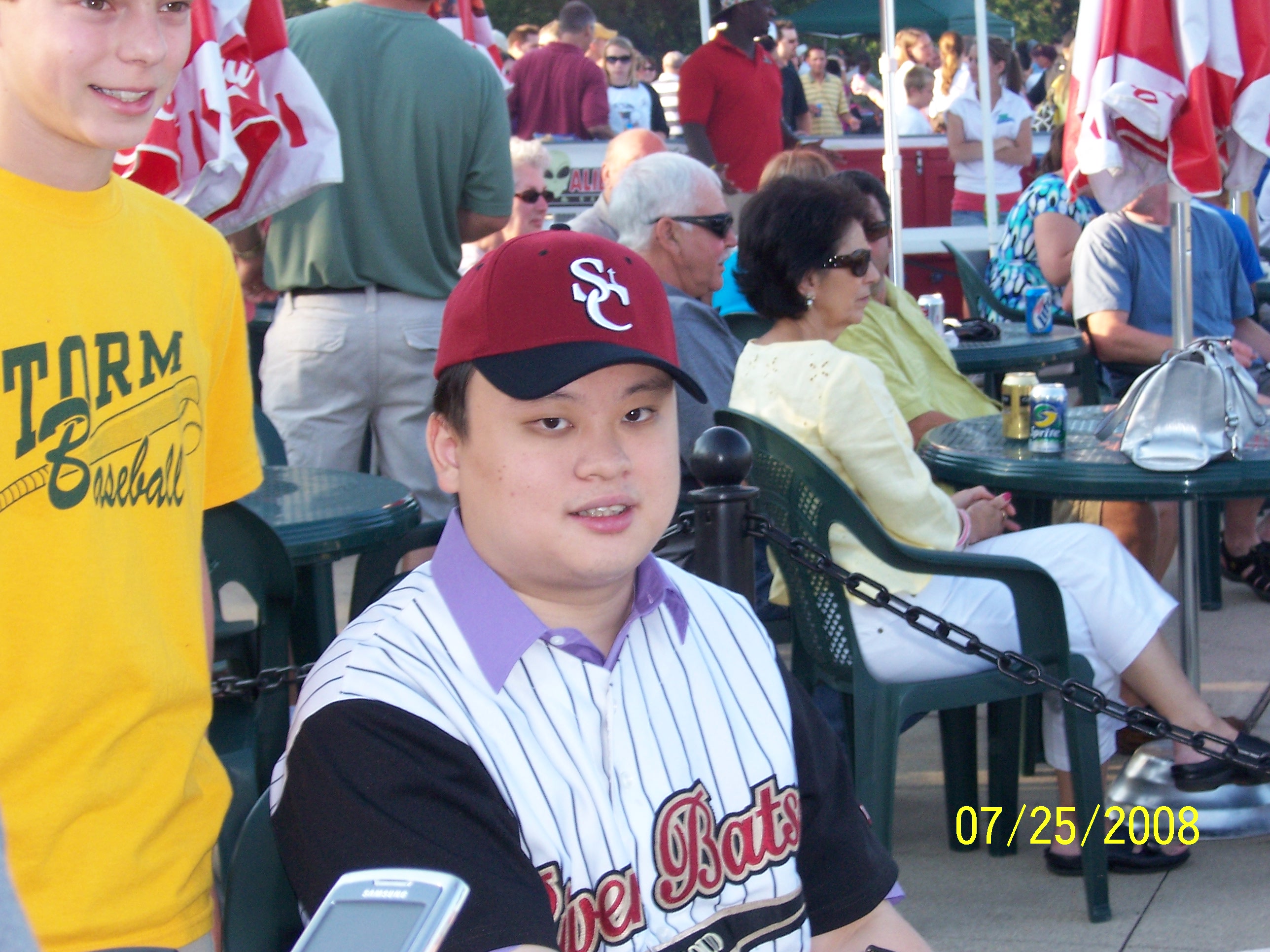The color photograph captures a lively outdoor event with numerous attendees seated at round dark green tables and green lawn chairs, some with drinks in front of them, suggesting a social gathering, possibly a baseball game or sporting event. In the foreground, there is a young boy of Asian descent, facing the camera with a slight smile. He is dressed in a distinctive outfit: a red baseball cap with a black brim and white "SC" letters, a purple button-down collared shirt underneath a pinstriped baseball jersey with black sleeves. The jersey prominently displays the word "BATS" in red text surrounded by black and gold. Next to him stands a young white male in a yellow t-shirt with blue text that reads "STORM BASEBALL" accompanied by a baseball graphic. The backdrop is filled with men and women sitting and standing, engaged in conversation. The image is bright and clear, taken outdoors during the daytime, with the date "07-25-2008" in yellow text at the bottom right corner.